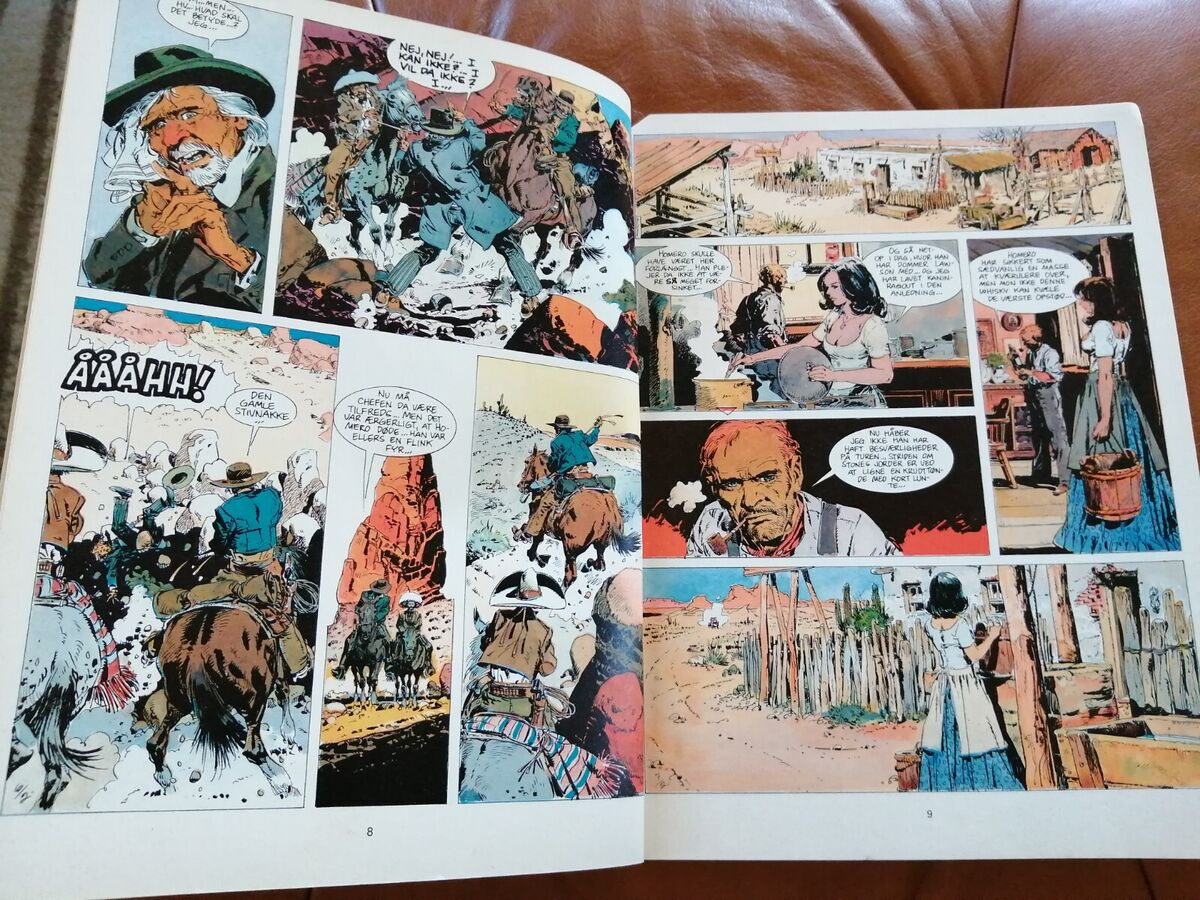The image depicts an open graphic novel resting on a brown leather couch, presenting both the left and right pages (pages 8 and 9). The comic, rendered in a detailed, realistic style, follows a Western theme. On the left-hand side (page 8), several panels feature an old man with a black hat, white hair, a white goatee, a white collared shirt, and a black overshirt, notable for his red nose. Adjacent scenes depict individuals riding horses against a desert backdrop with a large rock outcropping, suggesting a rugged frontier setting. Among these panels is a notable scene with a blue-shirted rider in a brown hat and another figure in a dark blue trench coat.

The right-hand side (page 9) transitions to a homestead environment, where the old man is seen returning home. A white adobe building and a red barn establish the setting. In subsequent panels, a dark-haired woman in a prairie blue dress, whose large breasts are halfway visible from her dress, is depicted. She appears in various scenarios: standing on a dirt road next to a wooden fence, holding a brown bucket, and most prominently, stirring a pot of food while conversing with a pipe-smoking man. This combination of domestic and frontier visuals encapsulates the essence of a bygone Western life, rich with narrative vignettes.